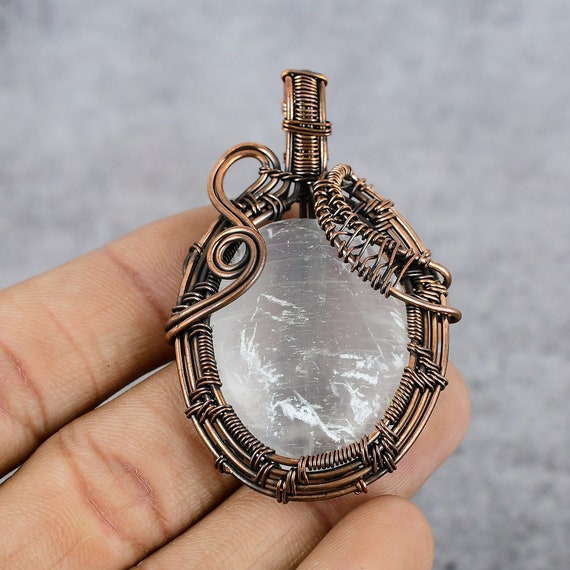This photograph depicts a left hand with four outstretched fingers—index, middle, ring, and pinky—holding a delicate pendant. The background is a fuzzy gray, designed to keep focus on the intricately detailed object. Centered in the image and resting on the fingertips, the pendant features an oval-shaped central element with the appearance of a scratched or scuffed white or gray stone, possibly quartz or moonstone. Surrounding this central stone is an ornate framework of twisted bronze or copper wire, forming elaborate coils and curves. The top of the pendant features a bottleneck-like design, with the wire coiling tighter around this area. The pendant, which might be part of a necklace, measures approximately two inches in height and about an inch to inch-and-a-quarter wide. The light complexion of the hand contrasts with the darker, time-worn metal of the pendant, highlighting the craftsmanship of the intricate wirework and the stone's subtle imperfections.